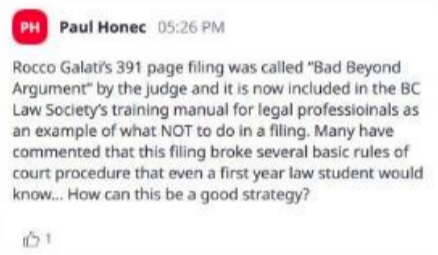The image depicts a social media post formatted in a square shape, reminiscent of those commonly found on platforms such as Facebook or Instagram. At the top of the post, there is a striking red logo displaying the initials "PH," representing the account owner, Paul Honeck. Below the logo, Paul's name is listed in bold black text, followed by the time of posting, "5:26 PM," rendered in grey.

The main body of the post consists of black text on a white background. It details a controversial filing by Rocco Galati, described by a judge as "bad beyond argument." The 391-page document has been incorporated into the BC Law Society's training manual for legal professionals as a cautionary example of poor legal practice. Comments on the filing highlight that it violated several fundamental court procedure rules, which are expected to be known even by first-year law students, questioning the efficacy of such a strategy.

At the bottom of the post, there is a grey thumbs-up emoji, indicating one like. Overall, the only color element on the page, other than the text itself, is the red "PH" logo, making it a visually straightforward yet detailed social media post.